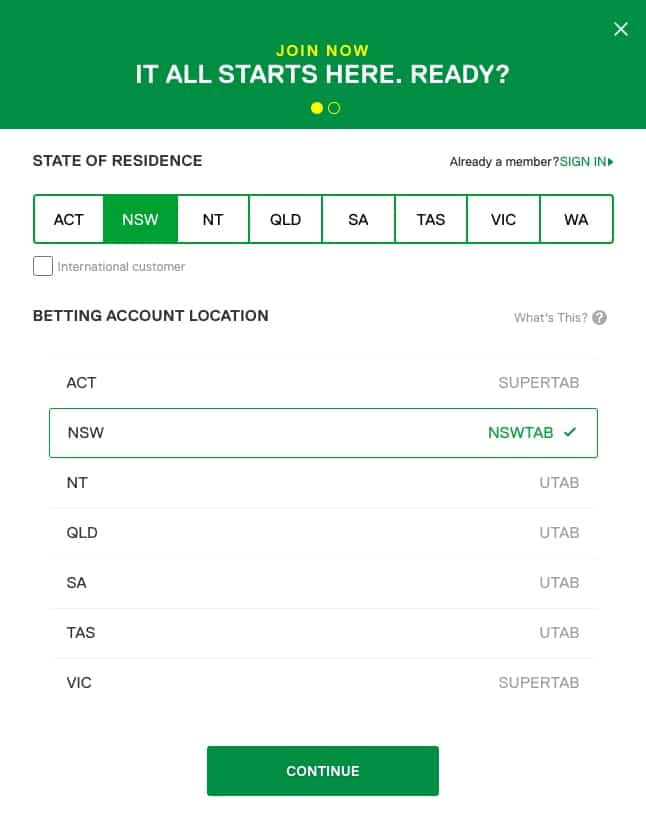The screenshot captures an application or website interface primarily focused on user registration or sign-in. At the top, a green banner with yellow text prompts, "Join Now," accompanied by a white tagline, "It all starts here. Ready?" with an 'X' button in the top right corner allowing users to close this prompt.

Beneath the banner, users are instructed to select their state of residence. The interface provides an option for existing members to sign in, marked by a hyperlinked "Sign In" text paired with a right-pointing arrow. 

The main content area features a horizontal series of green-bordered boxes representing different states. The box for "NSW" (New South Wales) is highlighted in green, signifying selection. The available states, listed from left to right, include: ACT, NSW, NT, QLD, SA, TAS, VIC, and WA.

Below these options, a grey checkbox labeled "International Customer" is available. Further down, users are informed about a "Betting Account Location," with a clarifying "What is this?" inquiry nearby.

The layout splits into two vertical columns, with options listed horizontally by layer. These include:

- ACT: Super TAB
- NSW: NSW TAB, highlighted with a green check mark and bordered
- NT: U TAB
- QLD: U TAB
- SA: U TAB
- TAS: U TAB
- VIC: Super TAB

At the bottom of the interface, a prominent green "Continue" button encourages users to proceed.